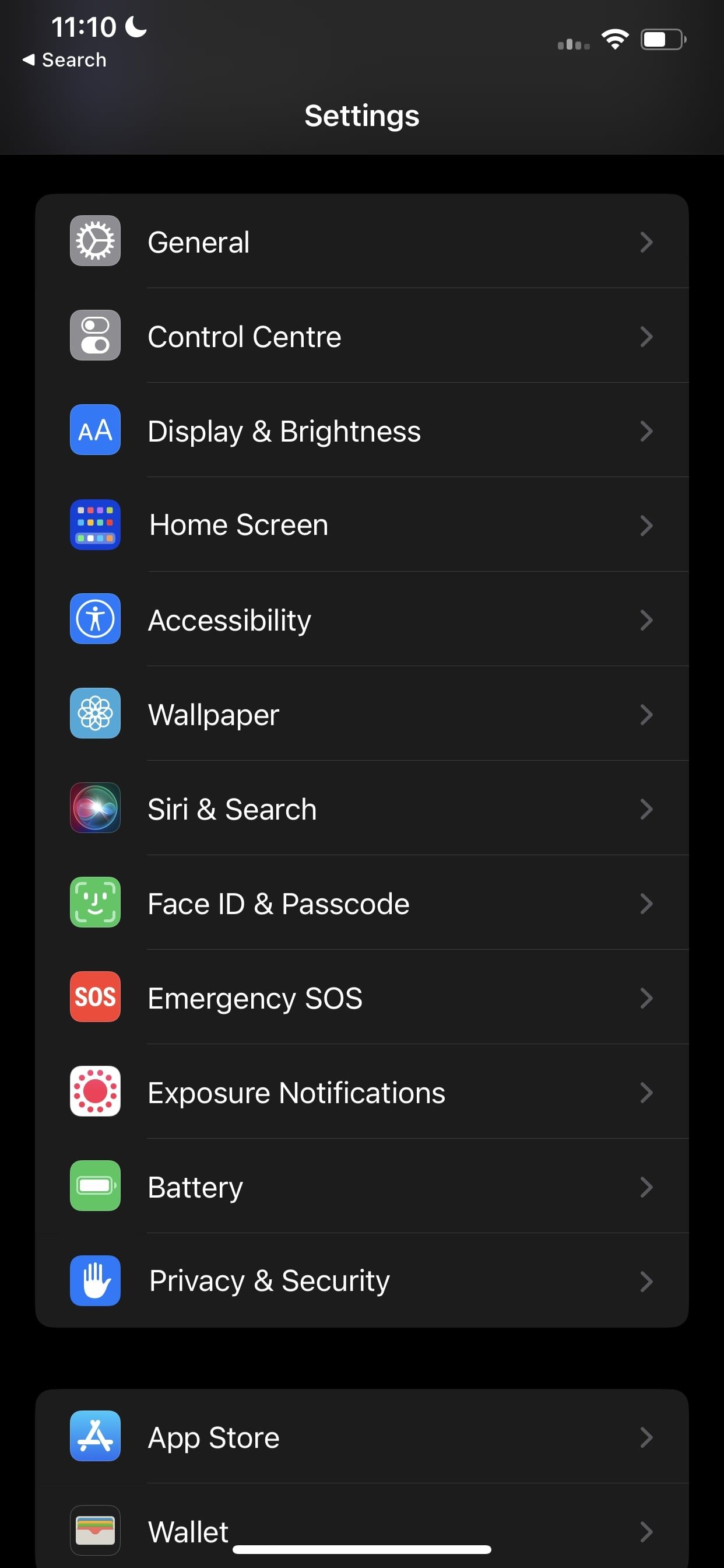A screenshot showcasing a dark-themed settings menu on a device. The top status bar indicates the time as 11:10 with the moon icon visible, suggesting it might be night mode or "Do Not Disturb" is enabled. In the upper left corner, there is a back arrow icon for navigation. The settings menu is listed on the screen with each item accompanied by a right-pointing arrow indicating further options. The listed settings include General, Control Center, Display & Brightness, Home Screen, Accessibility, Wallpaper, Siri & Search, Face ID & Passcode, Emergency SOS, Exposure Notifications, Battery, Privacy & Security. Further down, there's a separate section for the App Store and Wallet settings. At the bottom of the screen, a white bar is visible, typically indicative of gesture controls on modern smartphones.